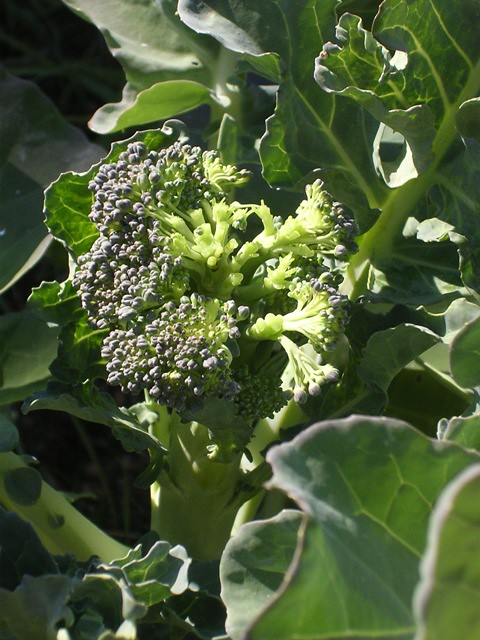A vivid close-up photograph captures the intricate details of broccoli or possibly broccolini plants growing outdoors. The sunny image highlights clusters of medium to dark green florets interspersed with distinctively darker, almost blue-green buds. Prominent, thick light green stems support the broccoli clusters, which are surrounded by large, wavy-edged leaves displaying a gradient from light green to dark grayish-blue. The foreground features slightly out-of-focus leaves with visible veins and indentations, adding to the textured complexity of the shot. The portrait orientation emphasizes the rich interplay of colors and the natural arrangement of the plant structure, creating a striking and detailed botanical study.